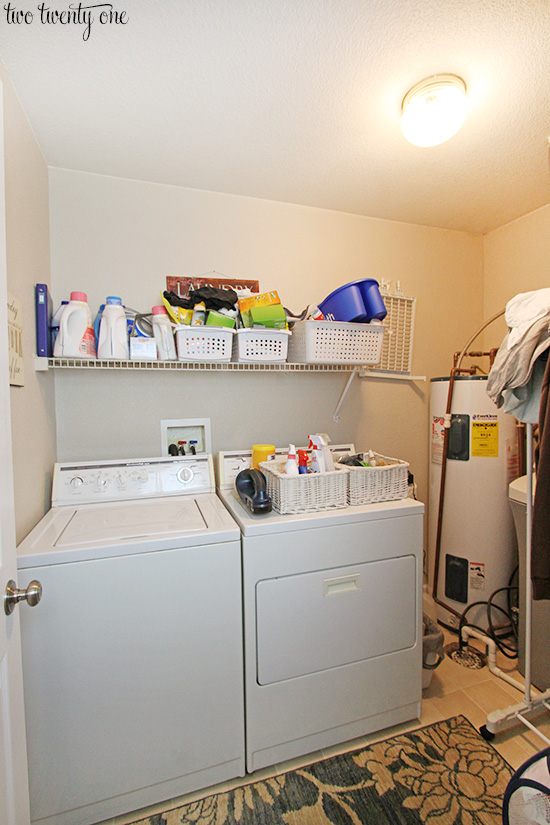The photograph captures a tidy home laundry room featuring a white top-loading washing machine to the left and a white front-loading dryer on the right. The room is predominantly white with touches of beige and blue, including a blue and beige rug with a floral pattern positioned in front of the appliances. A white wire shelf is mounted above the washer and dryer, holding a collection of baskets filled with various items, such as laundry detergent, spot remover, and other cleaning supplies. Additional baskets are situated on top of the dryer, containing laundry tape and spray bottles. In the background to the right, a water heater with hoses extends towards the wall. A barely visible rack with some shirts hanging on it can be seen off to the side, possibly used for folding or hanging clothes after washing. The room is well-lit by a flush mount ceiling light, and a somewhat hidden sign is placed behind the baskets on the shelf. The overall scene presents a well-organized and functional laundry space.